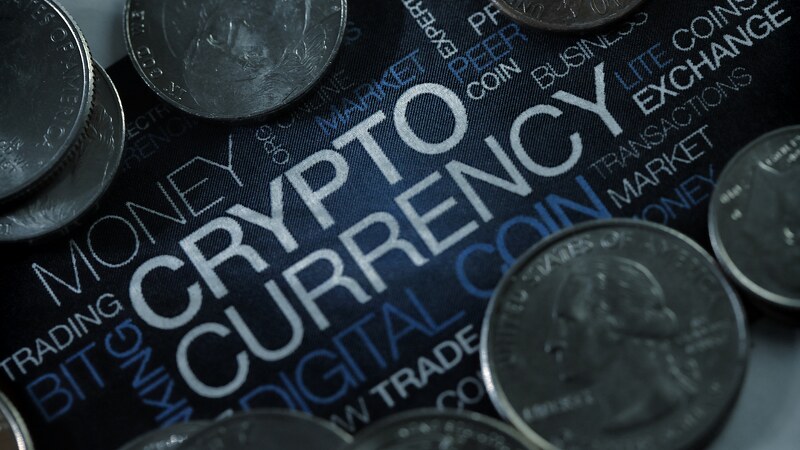The image features a textured navy cloth or possibly a dark-colored mouse pad, adorned with various words and phrases linked to finance in a mix of white, blue, and gray text. Key terms include “MONEY,” “CRYPTOCURRENCY,” “TRADING,” "BIT," "DIGITAL COIN," “MARKET,” "TRANSACTIONS," and "BUSINESS." Scattered across this backdrop are multiple silver coins, specifically quarters. There are two quarters on the right edge, three at the bottom, three in the top left with two partially stacked, and another one at the top right edge. These quarters appear as if they're slightly hovering, suggesting they're on a thick surface rather than directly on a table.